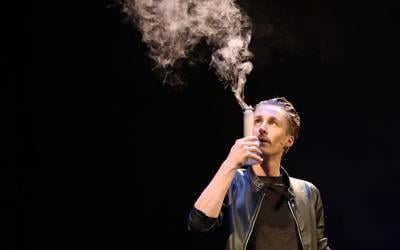In the image, a slender white male, possibly a performer or magician, is depicted against a pitch-black background, lending an air of mystery or drama. He stands slightly right of center, showcasing his upper body. His hair is slicked back, revealing dirty blonde or light brown strands, and he sports a brown mustache. Dressed in a black leather jacket with the sleeves casually pushed up, he wears a matching black shirt underneath. His right arm is bent at the elbow, holding a beige, cylindrical glass piece at face level. Wisps of smoke emerge from the top of this cylinder, forming a cloud above it. The man gazes intently at the rising smoke, adding a sense of intrigue to the scene. The entire setup, including his focused expression and the mysterious object, suggests he might be performing an illusion or scientific demonstration.